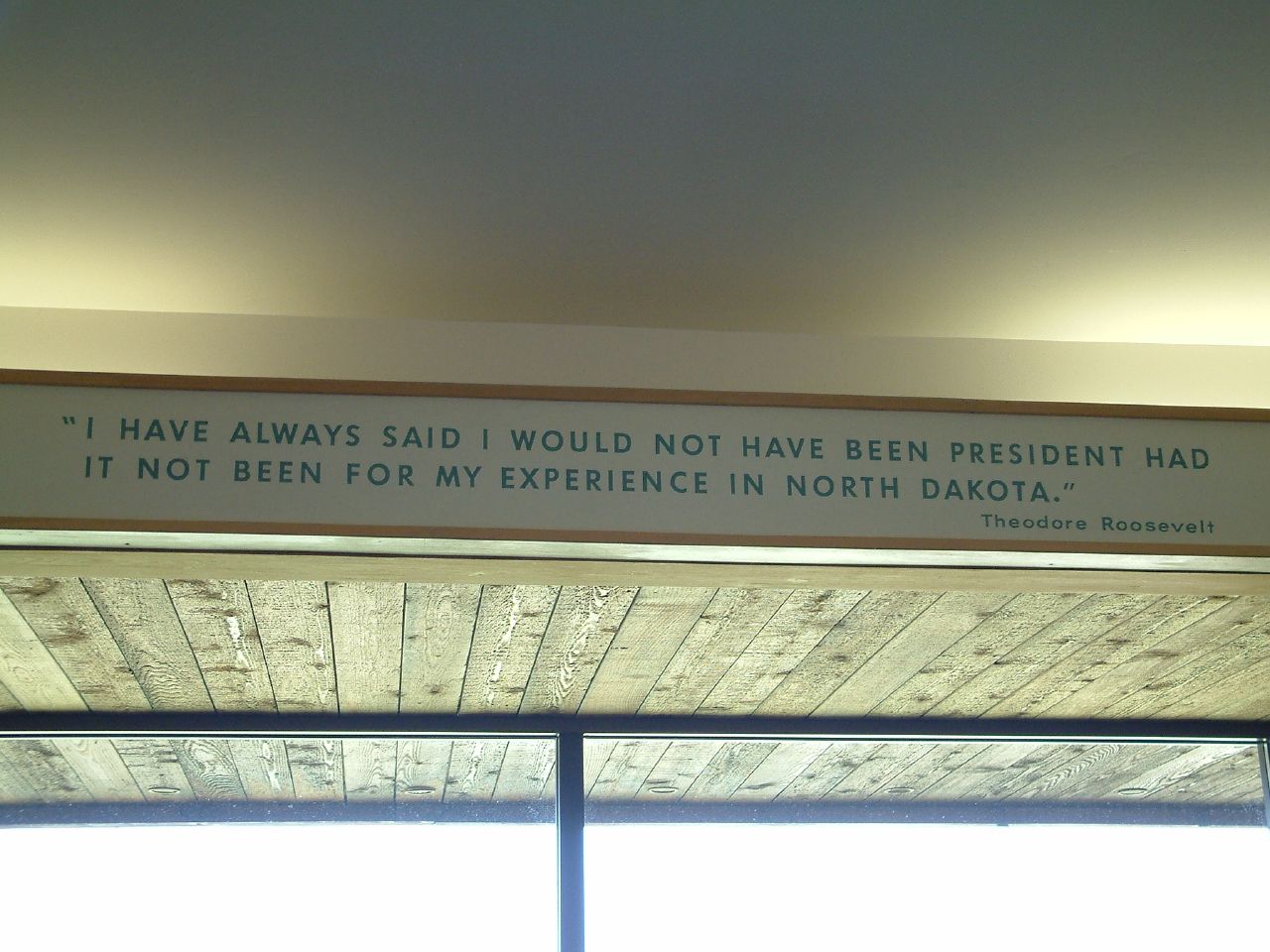This photograph showcases an inspirational quote displayed prominently above a large wooden-framed window, accentuated by a soft, backlit white and beige ceiling. The rectangular sign features a white background with sans serif text in blue, reading, "I have always said I would not have been president had it not been for my experience in North Dakota," attributed to Theodore Roosevelt. The sign is bordered in wood, and the scene captures the intricate detail of the wooden beams that support both the ceiling and the structure around the window. The image, taken at an upward angle, also reveals a portion of the wooden-paneled ceiling as seen through the window, emphasizing the architectural blend of wood and light within the space.